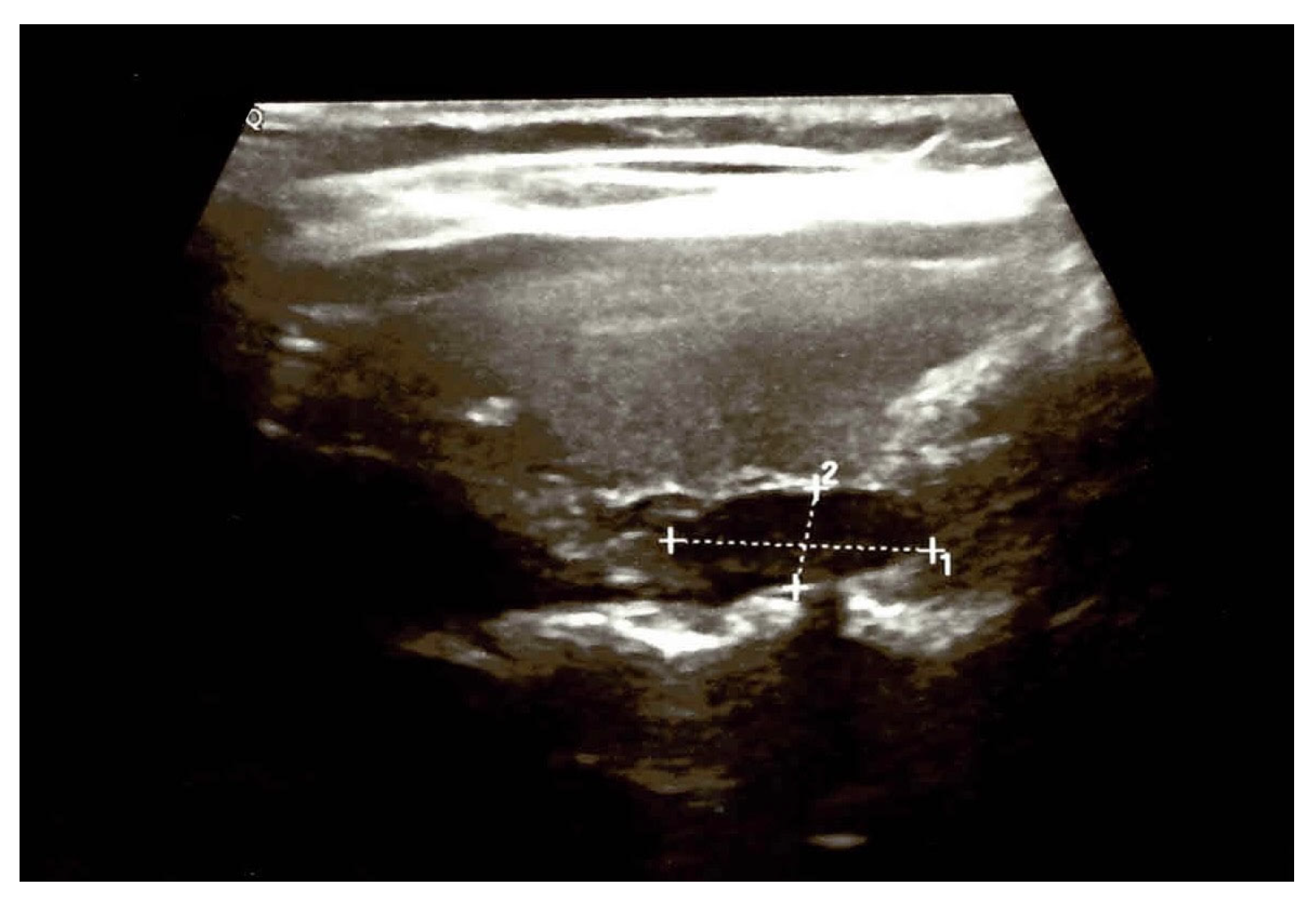The image appears to be an ultrasound, characterized by a dark black background with grainy details in varying shades of gray and white, typical of sonograms. At the center, there is an oval-shaped area, which is offset slightly to the right. The central area is intersected by two dotted lines forming a cross, with one line running horizontally and the other vertically. Each line has plus signs at both ends; the horizontal line is marked with "1" on the right end, and the vertical line with "2" at the top end. These lines seem to indicate measurements or points of interest within the ultrasound. The overall image is difficult to interpret clearly, and while it looks like it could be a medical scan typically associated with pregnancy, it's hard to determine what exactly is being shown, whether it's a baby or another object.